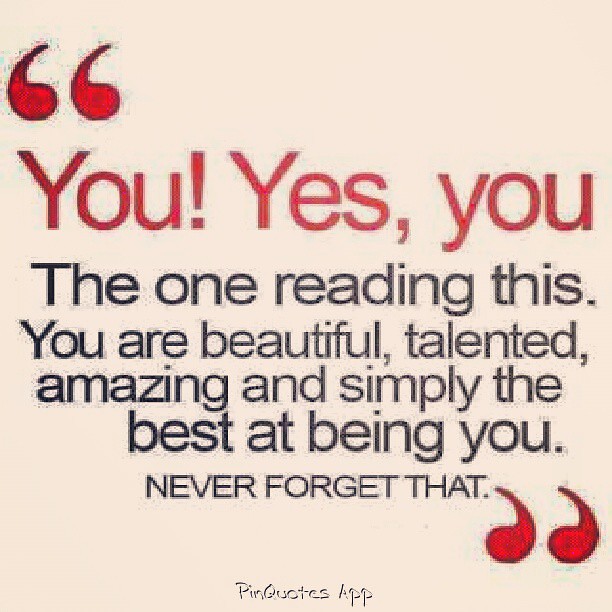The image features a square graphic with a light pink, almost off-white background. On this background, in the upper left corner, there are red quotation marks. Following this, a motivational message starts with the bold red text: "You! Yes, you." This is followed by a series of lines in black text which reads: "The one reading this, you are beautiful, talented, amazing, and simply the best at being you." The font varies slightly in size and weight, with "beautiful, talented, amazing, and simply the" appearing smaller than the other words. The message concludes with a bold uppercase statement: "NEVER FORGET THAT." Red quotation marks appear again at the end of the text. At the very bottom of the image, in light gray text, it says, "pin quotes app," indicating the source of the graphic.